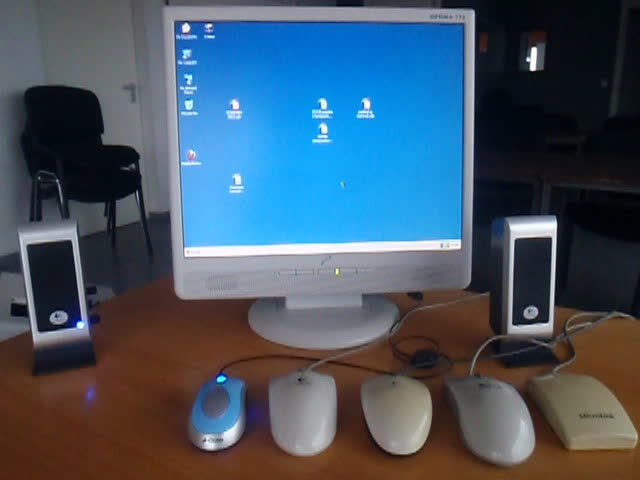The image depicts a retro computer setup from the early 2000s, prominently featuring a grey computer monitor displaying a blue screen with various icons, indicating it is likely running Windows 2000. Below the monitor are horizontal buttons and a green light. In front of the monitor on a brown wooden table lies an unusual arrangement of five computer mice; the first mouse on the left is blue with a matching blue light, followed by two white mice—one with a black cord, one with a grey cord—then a grey mouse, and finally another white mouse with a grey cord. Flanking the monitor are two silver speakers with black interiors and rotary dials, the left speaker notably illuminated by a blue light. In the background, a stack of black chairs is visible next to a white door with silver handles. The setup suggests an eclectic mix of old technology in a utilitarian space.